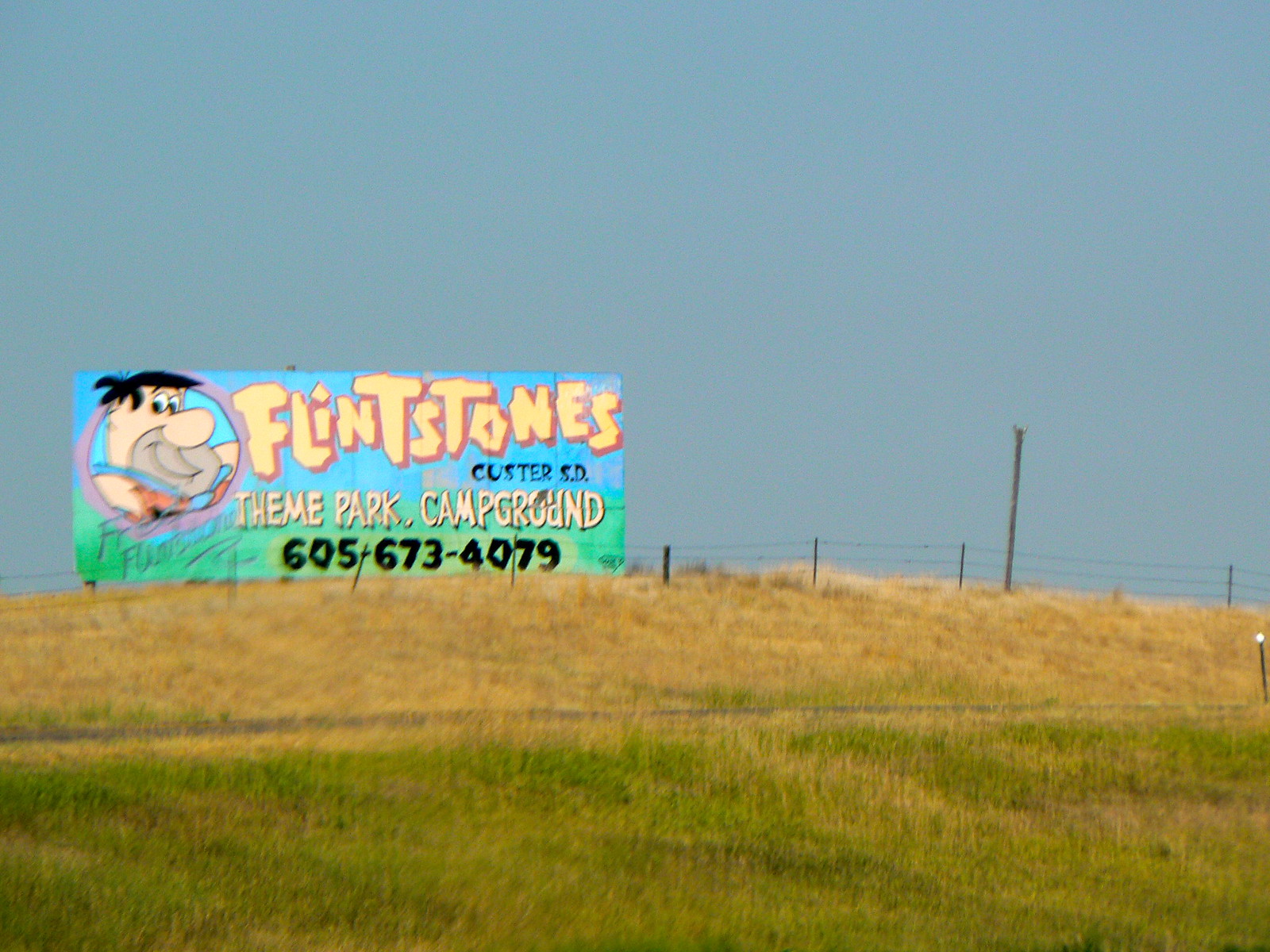This photograph captures a vibrant sign for the "Flintstones Cluster XD," a theme park campground, prominently situated beside a subtly sloping hill. In the foreground, patches of green and yellow grass dominate, leading up to a midway road that slices through the terrain. The grass transitions to a solid yellow hue further up the hill, culminating at a weathered barbed wire fence stretching the width of the image. Rustic wooden posts, rather than metal, support the fence, adding a rural charm.

Dominating the scene, the large, colorful sign features Fred Flintstone, offering a nostalgic appeal. The sign itself is divided: the top half bathed in blue, and the bottom half in green. "Flintstones" jumps out in bold orange letters, vividly contrasting the backdrop. Below, the readable contact number, 605-673-4079, invites visitors to explore the theme park campground. Looming above, the sky showcases a foreboding dark blue, hinting at impending rain and adding a dramatic contrast to the cheerful sign below.